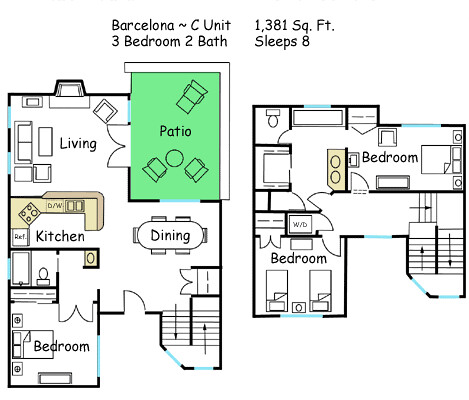This image is a detailed architectural floor plan of a house. At the top left, there is a legend featuring the title "Barcelona" followed by a distinctive tilde-like symbol. It identifies the house as "C Unit" and specifies that it contains three bedrooms and two bathrooms. On the top right, the legend notes that the house is 1381 square feet in size and can accommodate eight people.

The lower part of the image is split into two sets of floor plans, representing the first and second floors of the house. 

- **First Floor:**
  - The living room is located at the top left, furnished with sofas, chairs, a TV stand, and possibly a fireplace or a doorway leading to a patio.
  - Directly below the living room is the dining room, featuring a table surrounded by chairs.
  - To the left of the dining room is the kitchen, which is compact and designed in an L-shape.
  - Below the kitchen, a bathroom is depicted.
  - Adjacent to the bathroom is a bedroom.

- **Second Floor:**
  - Stairs lead up to the second floor.
  - This floor includes two bedrooms, one positioned at the top and another on the left side of the plan.

The clear labeling and careful arrangement of furniture and functional spaces make the floor plans informative and user-friendly.